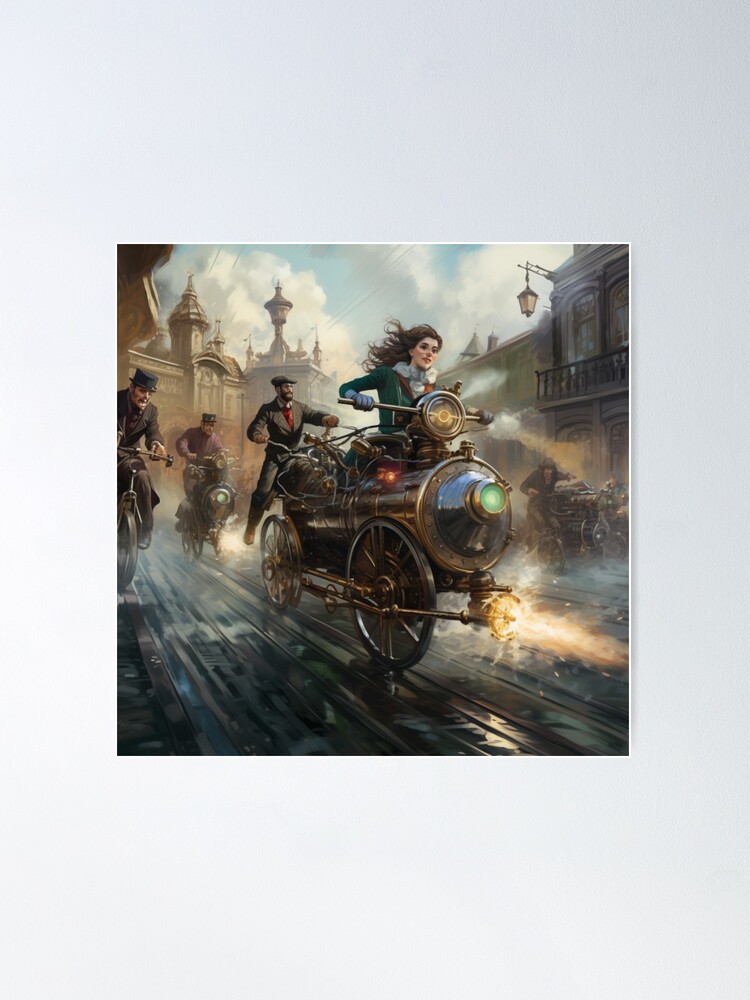The image is a detailed computer-generated artwork set against an off-white, grayish background. The focal point of the scene is a young woman with long, flowing brown hair, dressed in a green top paired with a white ruffly blouse and a jacket, giving off a Victorian vibe. She is riding a peculiar steam-powered vehicle that combines elements of a motorcycle and a train, featuring a cylindrical, gold-metal structure equipped with large black wheels with spokes, a green headlight in the front, and an additional light emitting an orange-yellowish glow, which appears almost like fire, from below. 

The vehicle has a unique design with handlebars and a gold steering mechanism. Behind her, three men adorned in Victorian-era outfits, including suits and hats—a top hat and caps—are pursuing her on similar contraptions. These men appear to be riding vehicles reminiscent of modified metal garbage cans with large wheels. The background showcases a cityscape with Victorian-style buildings embellished with spires, patios, and hanging lamps. The sky above is a vivid blue, dotted with fluffy white clouds, adding to the overall steampunk aesthetic of the piece. The artwork captures a blend of historical and fantastical elements, creating a whimsical yet nostalgic scene.